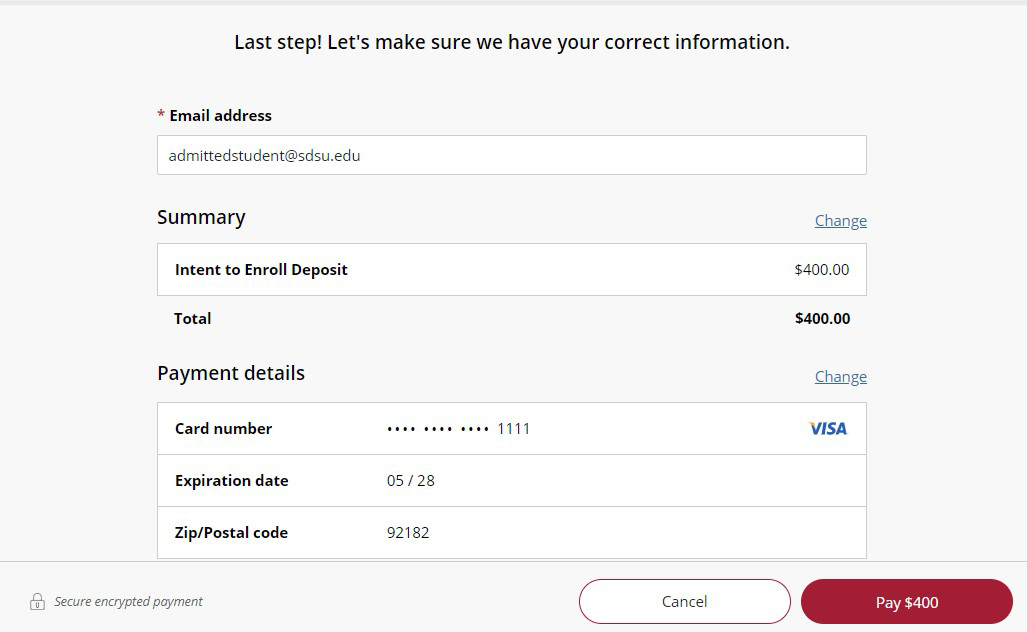**Detailed Caption:**

This image is a screenshot featuring a web page designed for a secure payment process. The background is a neutral grayish-white with predominantly black text, ensuring clarity and readability. 

At the top, a bold heading reads "Last Step!" emphasizing the importance of the current action, followed by "Let's make sure we have your correct information." Below, there is a field labeled "Email Address" marked with a red asterisk, indicating that it is a required field. The box contains the email address "admittedstudent@sdsu.edu."

Further down, there is a section labeled "Summary" in black font. Underneath, a clickable blue and underlined link says "Change." This section features a boxed breakdown of the financial details, highlighting an "Intent to Enroll Deposit" amounting to $400. Directly below, a "Total" is displayed prominently in bold black text as $400.

The next portion, labeled "Payment Details," comprises a series of white form fields. A blue "Change" link is adjacent to each field. The first field shows a partially obscured card number, revealing only the last four digits "1111," identified as a Visa card by the blue logo next to it. The expiration date is listed as "05/28," and the associated postal code is "92182."

At the bottom of the screen, a grey section labeled "Secure Encrypted Payment" features a padlock icon, symbolizing security. This section includes two buttons: a white "Cancel" button outlined in burgundy, and a prominent burgundy-red "Pay $400" button with white text, inviting the user to complete the transaction.

The image quality is crisp and clear, with well-balanced colors and a user-friendly, large font making it easy to read and navigate.